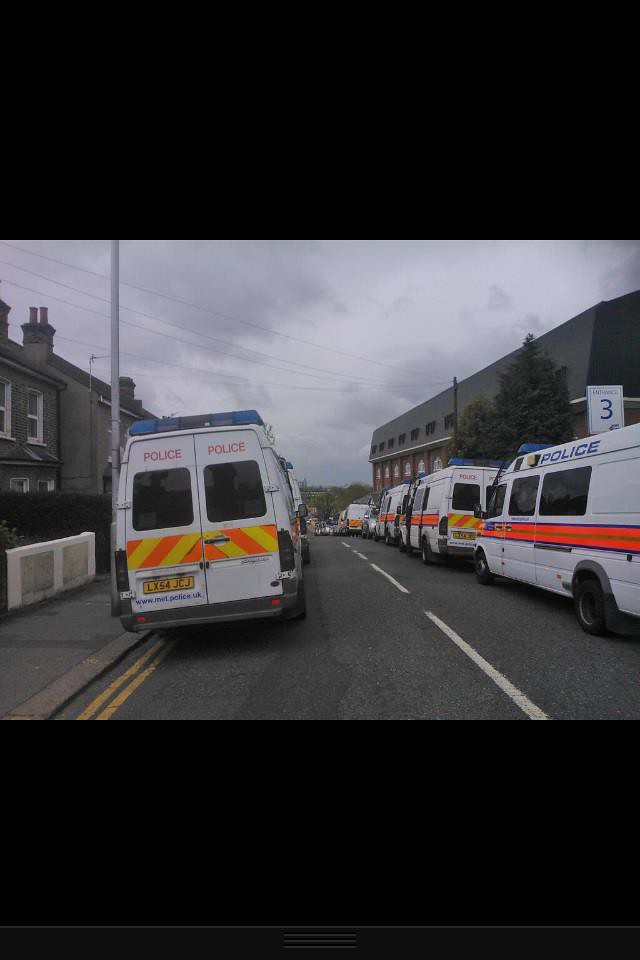This photograph, taken outdoors under an overcast sky with dark gray clouds, depicts a densely parked lineup of white police vans on both sides of a city street, possibly in the UK. Each van features a bright orange stripe running down the middle side and a pattern of orange and yellow diagonal chevrons on the back, along with the word "POLICE" in blue text. The vans are equipped with blue police lights atop their roofs and have very tinted windows. The one visible license plate reads "LX54 JCJ." On the left side of the image, there are multi-story gray brick buildings and a white fence, with a streetlight present. To the right, a multi-storied red-brick building with a dark roof is visible. The road itself is marked with thick white stripes in the middle and yellow stripes next to the curb. Above the vans on the right side, there's a sign with the number three. The composition of the image includes thick black borders above and below the cropped photograph.